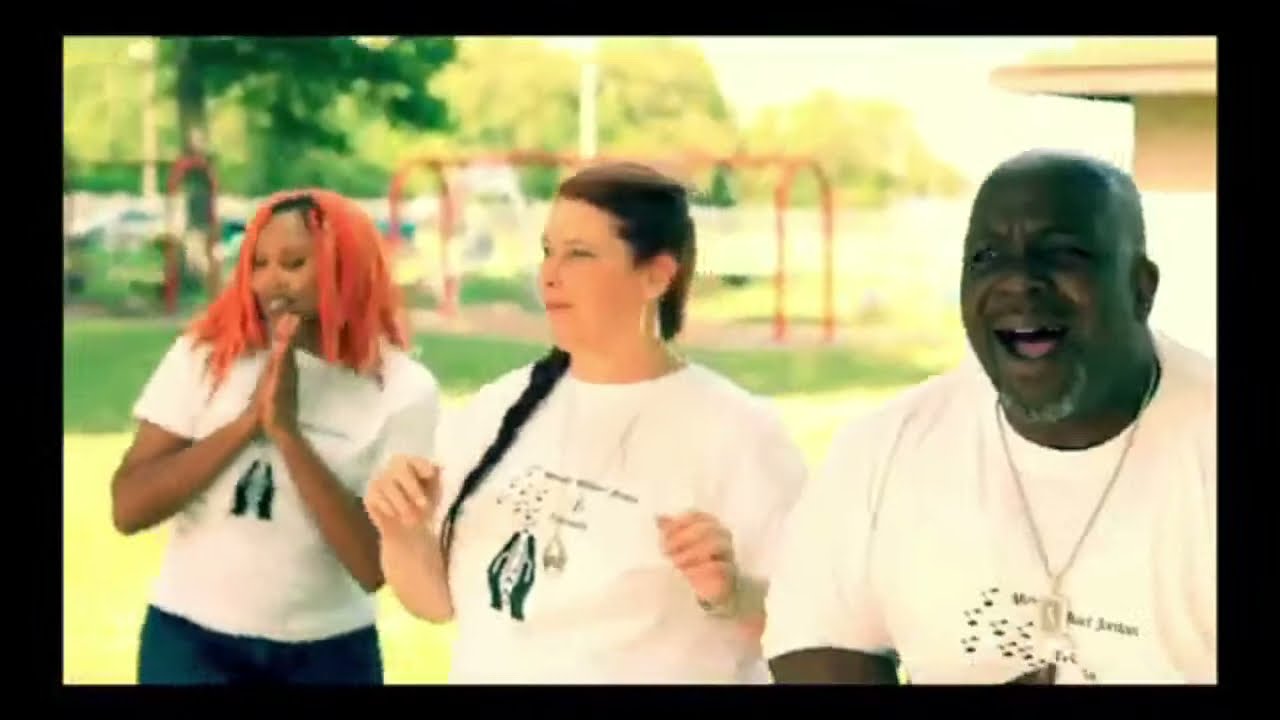Three people stand together, reacting excitedly to something off to the left, in what appears to be a park. On the left, there's a black woman with long, bright reddish-orange hair, wearing a white t-shirt adorned with a blurry design of praying black hands and text, and black jeans. She is smiling and holding her hands together in front of her, appearing to celebrate. In the middle is a Caucasian woman with brown hair tied into a long ponytail draped over her left shoulder. She wears the same white t-shirt and gold loop earrings, her hands poised at her sides as if about to pump them in the air. To the right stands a black man with a light gray goatee, also in the matching t-shirt, up to his chest visible. He is holding his stomach, mouth agape, as if in mid-laughter. Behind them is a green space featuring a tree with a red string or bar near the top left section, and a red swing set with visible bars. The overall mood is one of joy and surprise.